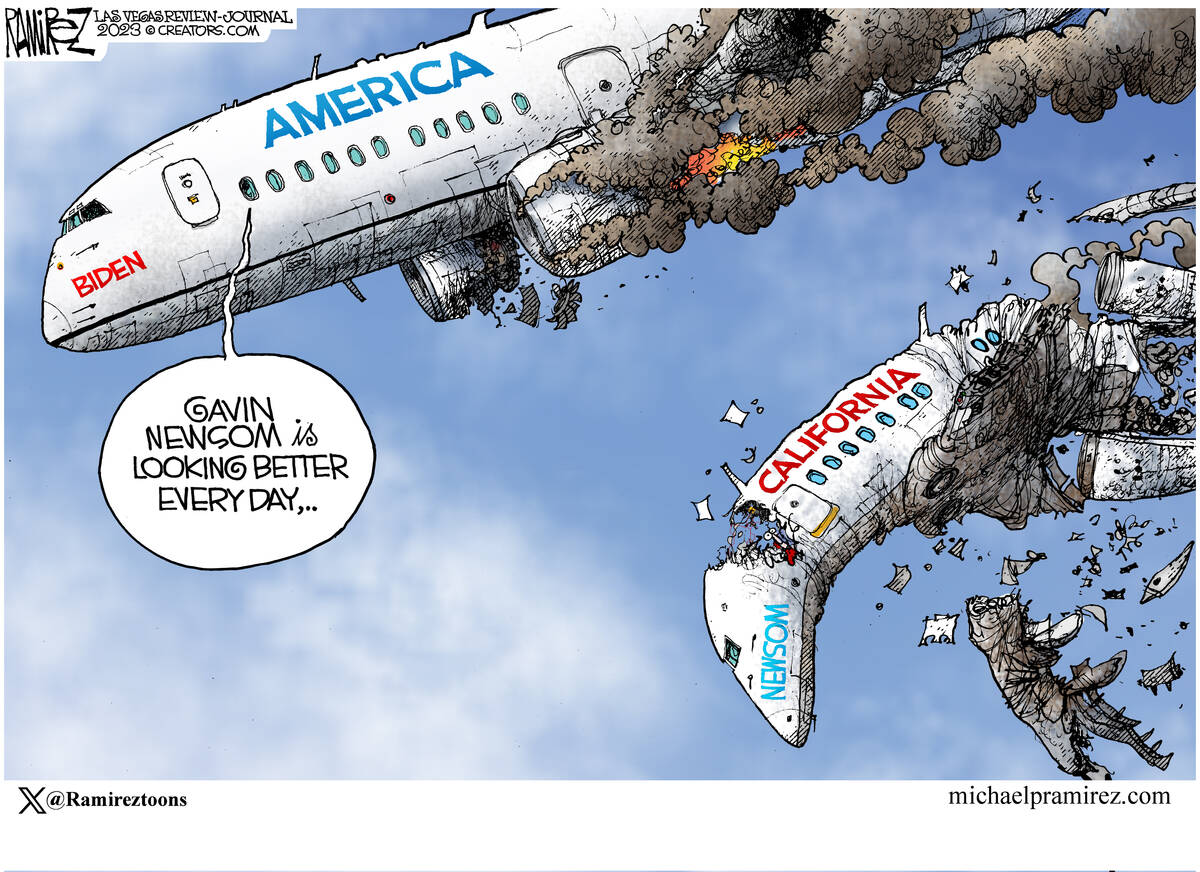The satirical cartoon by A. Ramirez, featured in the Las Vegas Review Journal 2023 and available on michaelpramirez.com, depicts two aeroplanes in crisis. The upper plane, labeled "America," is a large jumbo jet with its engines on fire but still mostly intact. The word "Biden" is written in red near the nose, and a speech bubble from the cockpit reads, "Gavin Newsom is looking better every day." Below this, a smaller, more severely damaged plane labeled "California" is depicted in a state of disintegration, with pieces breaking off and the structure on fire. The plane is marked with "Newsom" in blue on its side. The cartoon is credited to Ramirez with a watermark indicating the artist in the top left corner, and it includes a Twitter/X handle @RamirezTunes at the bottom. The artwork clearly portrays a political commentary on the states of America and California, underlining California's more catastrophic decline under Newsom with America following closely behind under Biden's leadership.